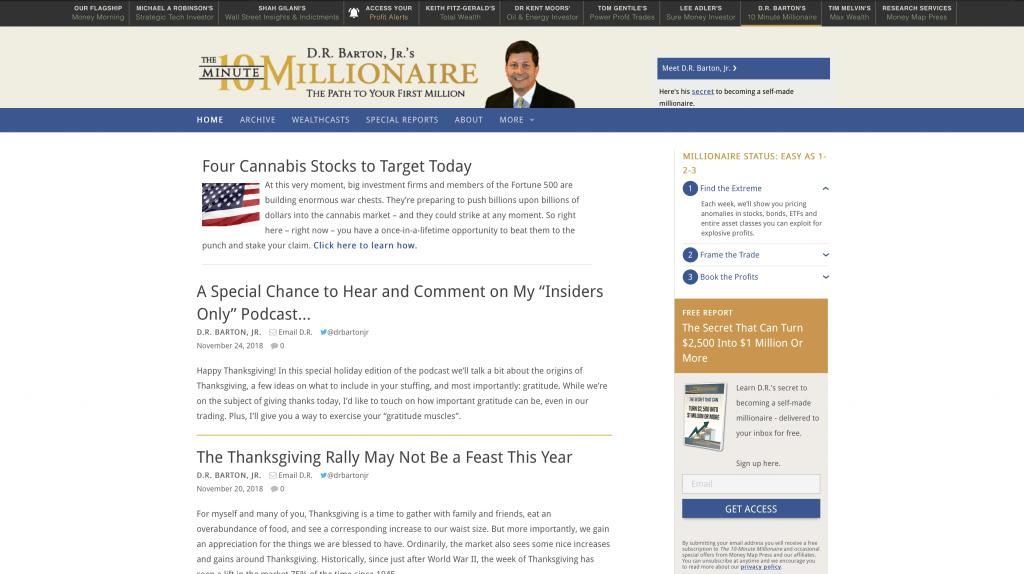Here is a detailed and cleaned-up descriptive caption based on the provided audio:

---

The image features a promotional advertisement by Dr. Barton Jr., renowned as the "10-Minute Millionaire," outlining a pathway to achieving your first million dollars. The central figure, Dr. Barton Jr., is depicted within a cream-colored box bordered by black on the top and blue on the bottom. An American flag is prominently displayed, and text indicates "Four Cannabis Stocks to Target Today."

The advertisement highlights a significant moment where major investment firms and Fortune 500 companies are amassing substantial funds, ready to invest billions into the burgeoning cannabis market. This presents a unique, once-in-a-lifetime opportunity for individuals to get ahead of these corporate giants and secure their own investment stakes.

The text urges viewers to "Click Here to Learn How," offering a special chance to access and comment on Dr. Barton Jr.'s exclusive insiders-only podcast. Another highlighted section states, "The Thanksgiving Rally May Not Be a Feast This Year," though the specific year is not mentioned.

On the side of the image, a step-by-step guide to attaining millionaire status is presented: 
1. Find the Extreme
2. Frame the Trade
3. Book the Profits

Beneath this guide, there is a free report titled "The Secret That Can Turn $2,500 Into $1,000,000 or More." It encourages users to learn Dr. Barton's secret to becoming a self-made millionaire by signing up to receive the report in their inbox for free. An email sign-up box is provided with a call-to-action button labeled "Get Access."

---

This caption captures the essence and details of the advertisement effectively.